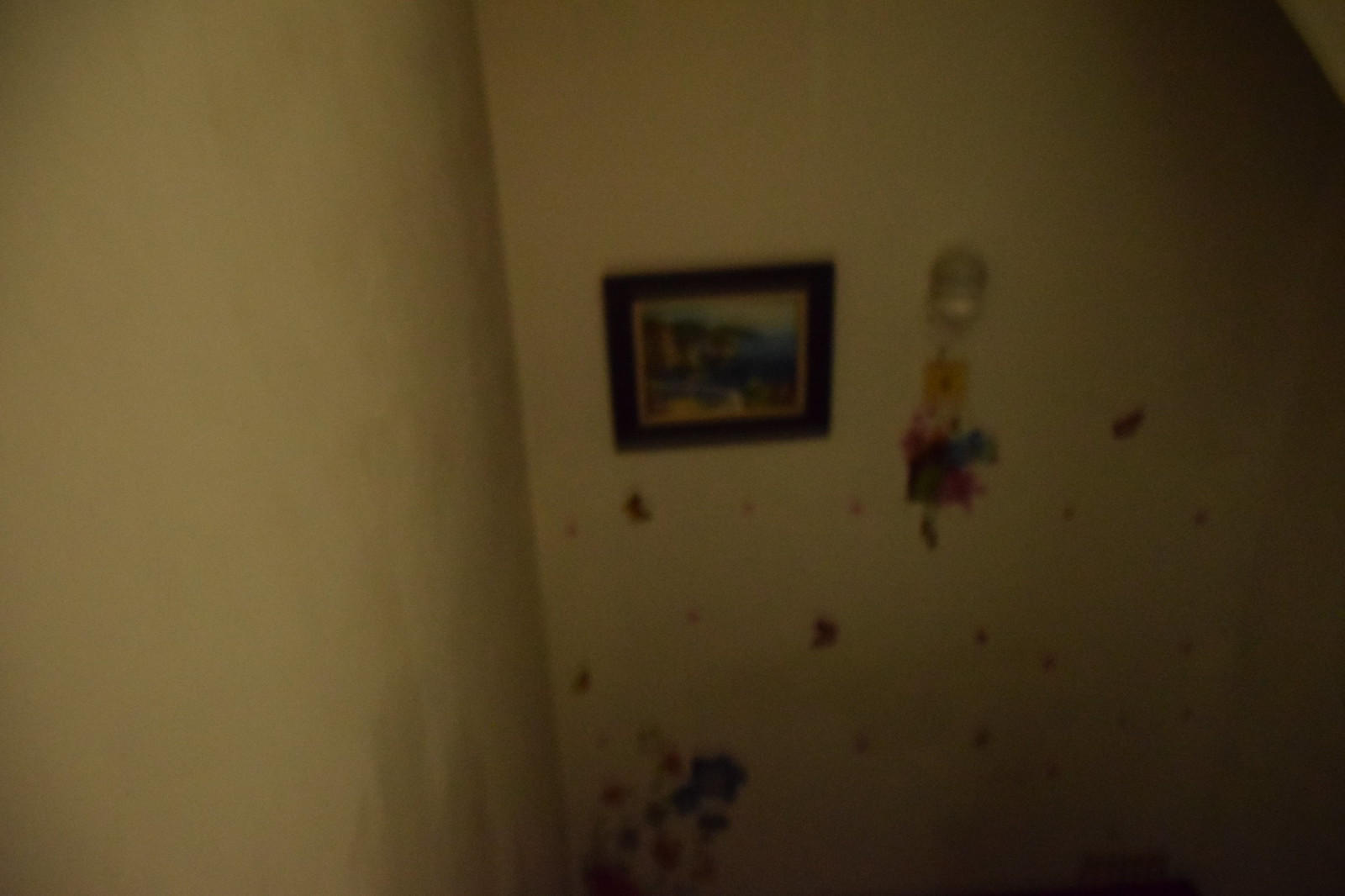The image depicts a dimly lit, aged interior with white walls that intersect at the back. Dominating the background is a square picture frame with a dark border, though the details within the frame are indiscernible. The walls themselves appear to be splattered with various marks and stains, suggesting objects might have been hurled against them. Collectively, these marks extend from the lower left upward, particularly concentrated near the frame. To the right of the visible picture frame (or the left from the viewer's perspective), there seems to be another object hanging, though its exact nature remains unclear. The overall impression is one of neglect, with the walls appearing dirty and cluttered.